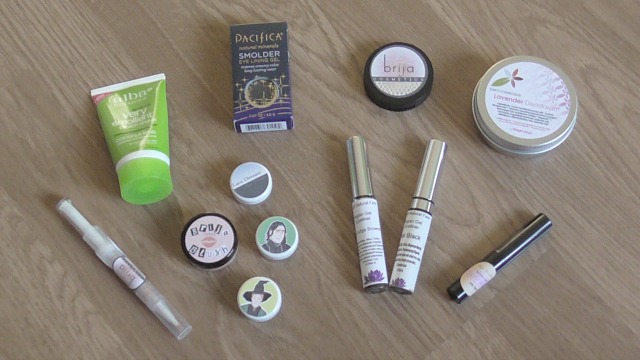This landscape-oriented photograph showcases a close-up of a modern wooden table, crafted in a pale butcher block style characterized by its varied wood patterns. The table is adorned with an assortment of cosmetics from different brands, predominantly featuring items from the brand "BRIJA," spelled B-R-I-J-A.

Starting from the left, there's a long tube, potentially a lip dye or gloss applicator. Next to it is a short, toothpaste-like tube from ALBA, labeled as a very exfoliant cream, colored in bright green with a matching cap. To the right of these are four small cylindrical containers, likely holding lip glosses, powders, or rouges. One container features a character resembling Professor Snape from Harry Potter, set against a green background, while another depicts a witch with a yellow background. Additionally, there's a pink-backgrounded cylinder labeled "Bria Blush," with block letters styled like magazine cutouts, and an image of lips, indicating it might contain lip gloss.

Above these items, there's a boxed item labeled "Pacifica Smolder," which appears to be eye shadow, though the writing is largely illegible apart from a visible barcode on the bottom. Next to this is another BRIJA product in a flat cylindrical form. Further along is a larger tin labeled "lavender something," adorned with a flower illustration and housed in a white background with extensive, hard-to-read text.

Below these items are two applicators, possibly mascaras, marked with the word "black" and decorated with small purple flowers. Their extensive text makes them difficult to read. Finally, there is a black cylindrical object, potentially a lipstick or eyeliner, entirely black with a pale peach label featuring additional, unreadable writing.